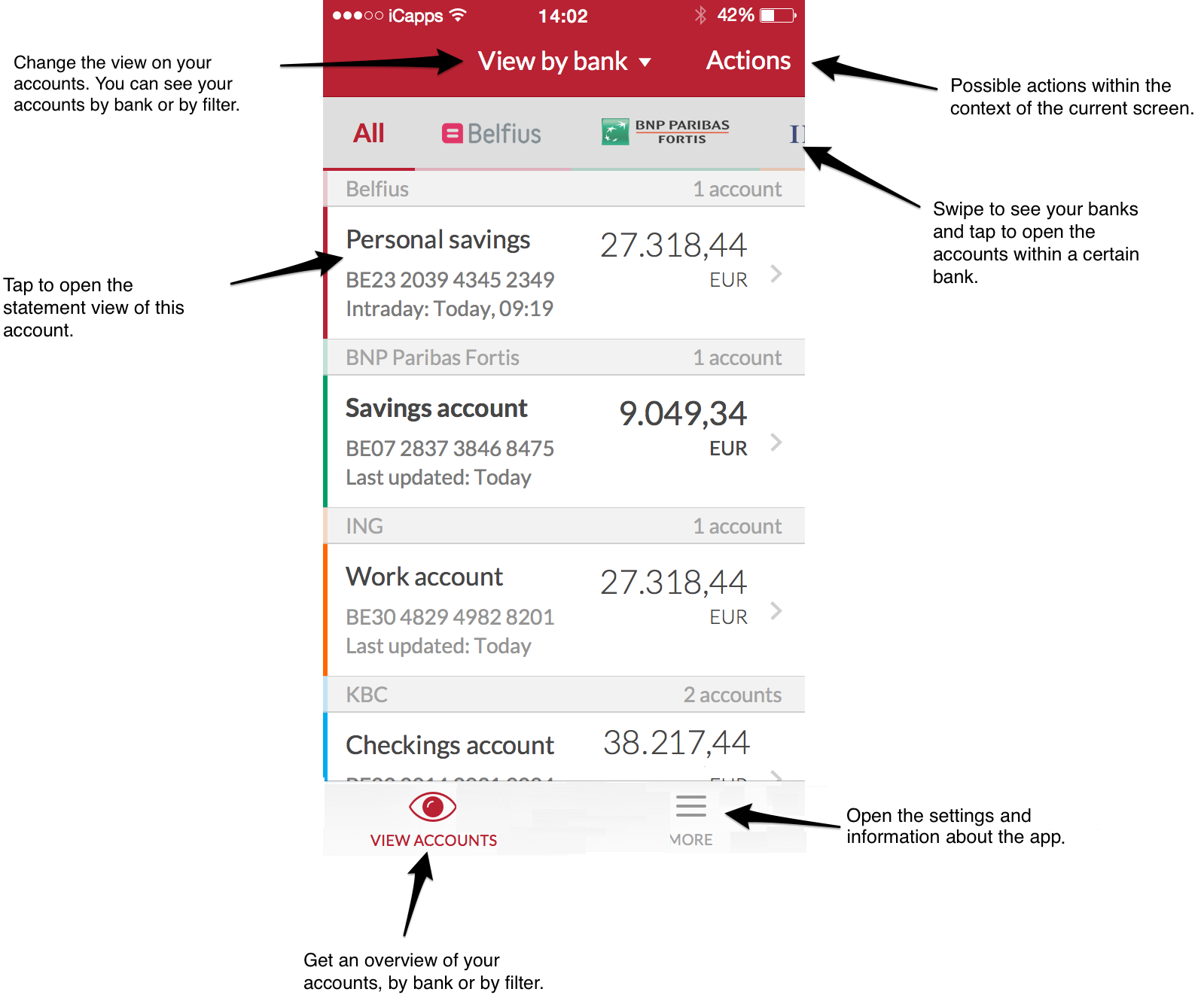**Caption: Detailed Screen Guide Demonstration for Banking App**

The edited screenshot showcases a banking application interface, captured on a mobile device, evident from the layout and navigation icons typical of smartphones or tablets. 

In the top-left corner of the screen, three out of five white ellipses indicate the cellphone signal strength, accompanied by a capital letter "I" with "CAPS" in small text and a Wi-Fi symbol. Centrally at the top, the time is displayed in military format as 14:04, alongside a grayed-out Bluetooth icon and a battery indicator showing 42%.

Below this status bar, the central section reads "View My Bank" with a dropdown arrow to its right. To the right side, there is a label "Actions" with a black arrow directing attention to it. Below "Actions," black text in a white box explains possible actions within the current screen context.

On the left, another black arrow points to "View My Bank," accompanied by text explaining that users can change their account view by bank or filter. Just below, a gray rectangle with a corresponding arrow instructs users to swipe to see their banks and tap to access accounts within a selected bank. The word "All" is highlighted in red within this dark gray rectangle, indicating the selected view.

Adjacent to "All," a hot pink square with gray lines and text reads "Belfius." Another square in dark green with white stars and text states "PNP Paribas Fortis," with a red underline. Multiple sliding rectangles below represent various accounts:

1. **Belfius**: Mid-gray background with dark gray text indicating "1 account." A black arrow points to this section, explaining tapping will open the account's statement view. It lists "Personal Savings" in bold black with a balance of €27,318.44. Further details include the account number "BE23203943452349" and the latest update date "09...19."

2. **PNP Paribas Fortis**: Similar setup with bold "Savings Account" showing €9,049.34, marked by a green line. The account number "BE07283738468475" and last update "today" are shown.

3. **ING**: This section has an orange line, indicating "1 account" labelled "Work Account" with a balance of €27,318.44. Details include "BE3048299828201" and "last update today."

4. **KBC**: Featuring a blue line and "2 accounts," it highlights a "Checking Account" with €38,217.44. A red "i" symbol invites users to "View Account," with a corresponding arrow explaining how to get an overview of accounts by bank or filter.

A "More" icon consisting of three black lines and the label "More" is on the right. A black arrow indicates this opens the settings and provides app information.

This caption comprehensively describes a screenshot from a mobile banking app, emphasizing navigation cues, account details, and user instructions.